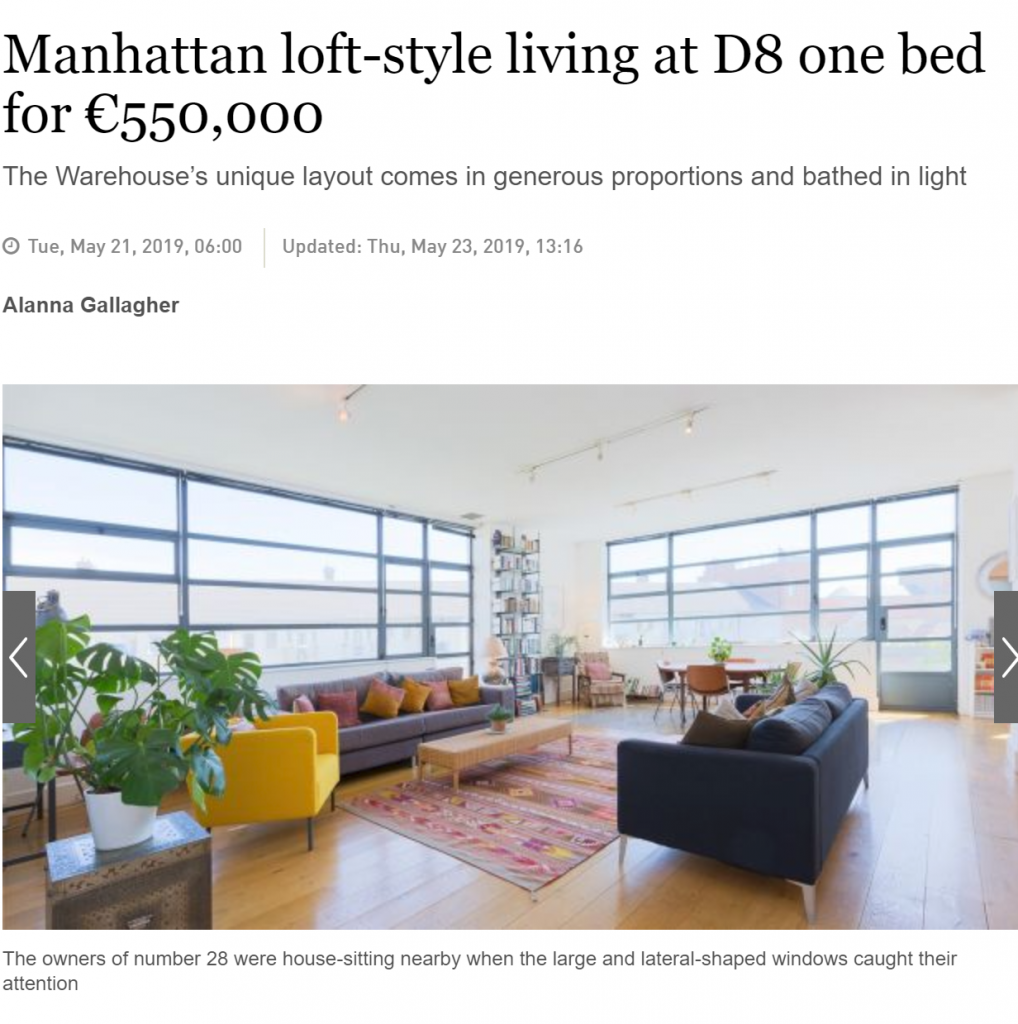This image is a screenshot from a website showcasing a stunning Manhattan loft-style apartment. The webpage features a large photo of the apartment at the bottom, set against a clean white background. At the top, a prominent headline in dark gray reads: "Manhattan Loft Style Living at £D8 - One Bed for $550,000." Below the headline, a subheading elaborates: "The warehouse's unique layout comes in generous proportions and bathed in light." The post was originally made on Tuesday, May 21, 2019, and updated on Thursday, May 23, 2019. 

The photo features a view of the apartment's living room, captured from a corner angle. It highlights two sides with very large windows that offer a stunning view of the cityscape outside. Inside, the room boasts beautiful hardwood flooring and elegant furnishings. The center of the living room is adorned with a rug featuring Native American motifs, flanked by two sofas — one lighter and one darker in color. Additionally, a very large green plant, identified as a philodendron, adds a touch of nature to the left side of the room.